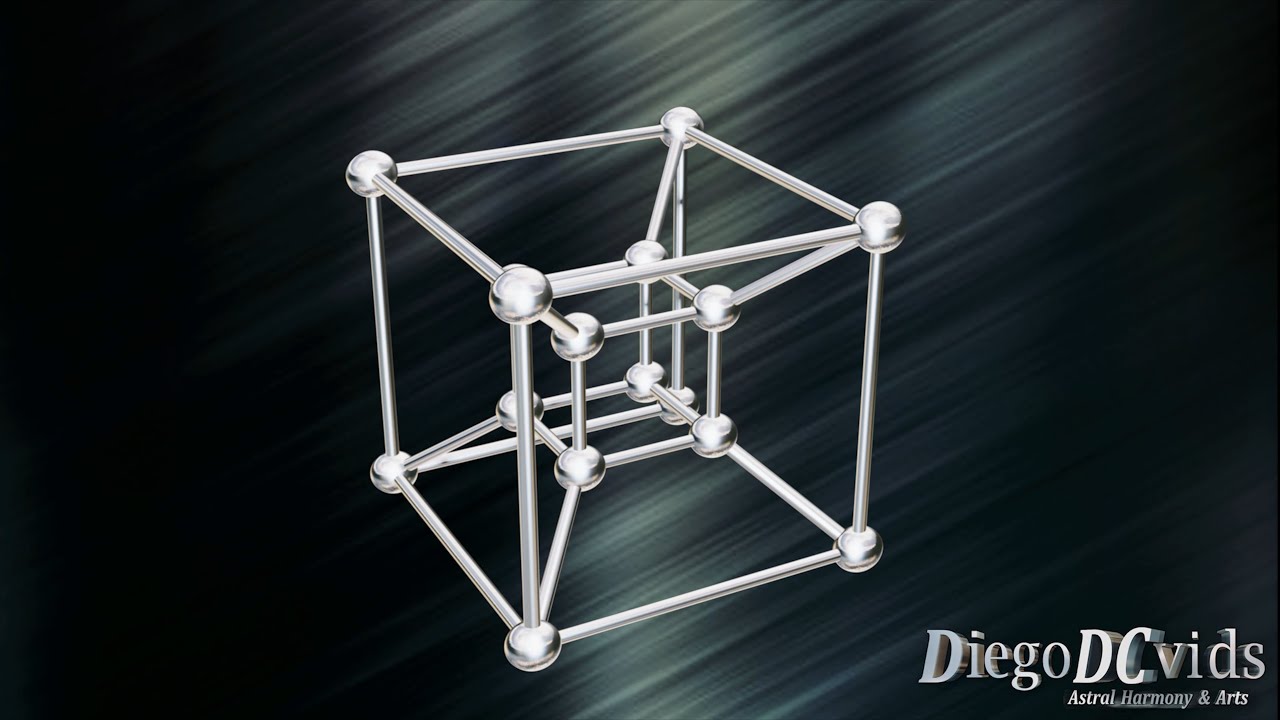The image showcases a piece of digital art featuring a three-dimensional cube structure. The main cube is constructed from silver metallic rods with spherical nodes at each corner. This outer framework contains a smaller inner cube formed in the same manner, creating an intricate and layered appearance. The artwork gives a molecular vibe due to its geometric precision. The background is predominantly black, interspersed with subtle whitish-gray streaks running diagonally from the top right to the bottom left, adding depth and contrast to the scene. In the bottom right corner, there is a metallic-looking text logo that reads "Diego DC Vids," with "Astral Harmony & Arts" inscribed below in smaller letters.